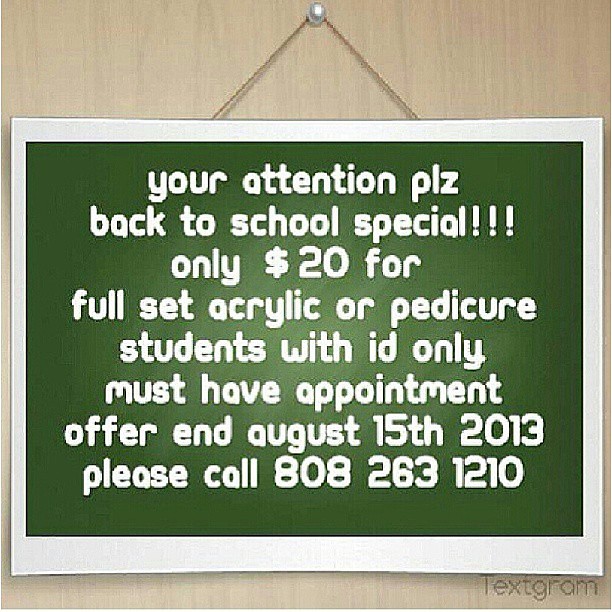The image features a computer-generated design resembling a square sheet of printer-sized paper hung on a wood-grain background, evoking the look of a notice pinned to a wall or door. The wood grain is depicted in light beige to grayish-brown tones. The "paper" has a white border framing a green background, giving the appearance of being secured by twine and a silver thumbtack. The white text on the green background announces: "Your Attention Please (PLZ). Back to School Special!!! Only $20 for a Full Set Acrylic or Pedicure. Students with ID Only. Must Have Appointment. Offer Ends August 15, 2013. Please Call 808-263-1210." At the bottom right corner, beneath the main content, the word "textgram" is visible, indicating the use of the Textgram app for creating the image.